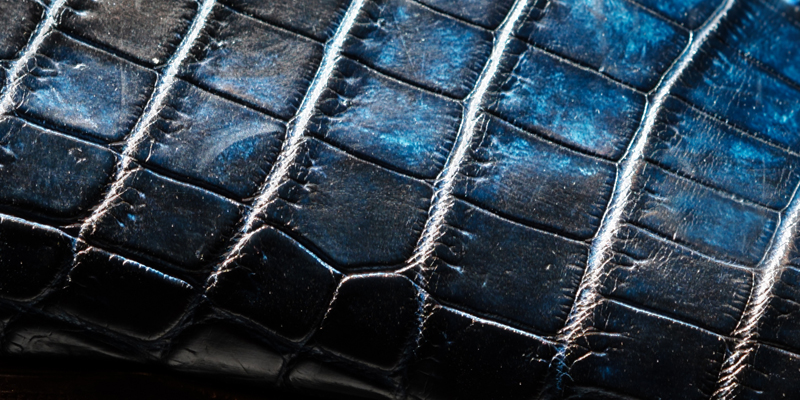The image is a very close-up photograph of a scaly, deeply embossed fabric or material, possibly crocodile skin leather that has been dyed a deep blue to almost black. The surface has a reflective quality and features a complex pattern of vertical and horizontal lines, creating rectangular shapes across multiple layers. The ridges are pronounced, giving the material a tactile, textured appearance. In the upper and right portions of the image, the rectangles are uniform, while towards the bottom they become less consistent, almost merging together. The precise type of object covered in this material is indistinguishable due to the close-up nature of the shot, but the detailed creasing and embossing suggest it could belong to an accessory like a shoe or a purse.